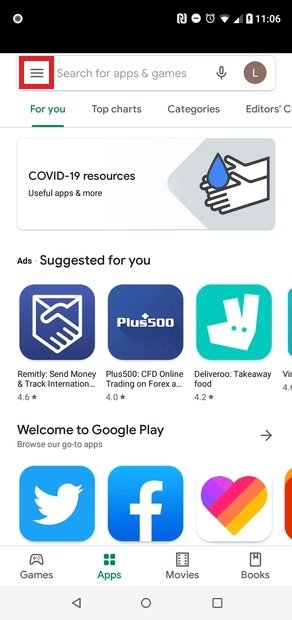This detailed caption captures all the elements described in the screenshot of the Android device showing the Google Play Store app:

---

Screenshot of the Google Play Store on an Android device. 

**Top Bar Icons:**
- Notifications: There's a small notification circle at the top left and another notification that looks like an "R" and "J" connected.
- Status Indicators: A "Do Not Disturb" icon, an alarm icon, nearly full Wi-Fi signal, and half-full cellular signal. The battery is fully charged, timestamped at 11:06.

**Highlighted Feature:**
- A red square highlights the hamburger icon, indicating where you can search for more menu options.

**Search and User Profile:**
- Search Bar: Allows searches for apps and games, and includes a microphone icon for voice searches.
- User Profile: The user is signed in but has not customized their avatar; it is a default grayish-brown circle with a white "L".

**Main Sections and Tabs:**
- Currently Selected: "For you," highlighted in green.
- Other Tabs: "Top charts," "Categories," and what appears to be "Editor's choice" (abbreviated as "Editor C").
  
**Content and Suggestions:**
- COVID-19 Resources: Includes useful apps featuring an image of someone washing their hands with a water drop.
- Ads: 
  - An app showing two people holding hands.
  - "Remitly: Send money and track international..." (trails off), rated 4.6 stars.
  - A blue square with the label "Plus 500, Plus 500: CFD online trading on Forex..." (trails off), rated 4.0 stars.
  - An icon showing bunny ears with fingers, related to "Deliveroo: Takeaway food," rated 4.2 stars.

**Welcoming Information:**
- Heading: "Welcome to Google Play."
- Subheading: "Browse our go-to apps."

**Highlighted Apps:**
- Twitter: Icon of a white bird in a blue square.
- Facebook: Icon of a white "F" in a blue square.
- An app icon with a rainbow-colored heart (purple, red, orange, yellow) in a white square.
- Another app whose icon is cut off.

**Navigation and Instruction:**
- Bottom of Screenshot: Google menu options with icons - a left arrow, a circle, and a square.
- The user seems to be guided on "How to find the menu button in the Google Play app store."

---

This descriptive caption fully reflects the details in the original voice-generated description, organized for clarity and thoroughness.